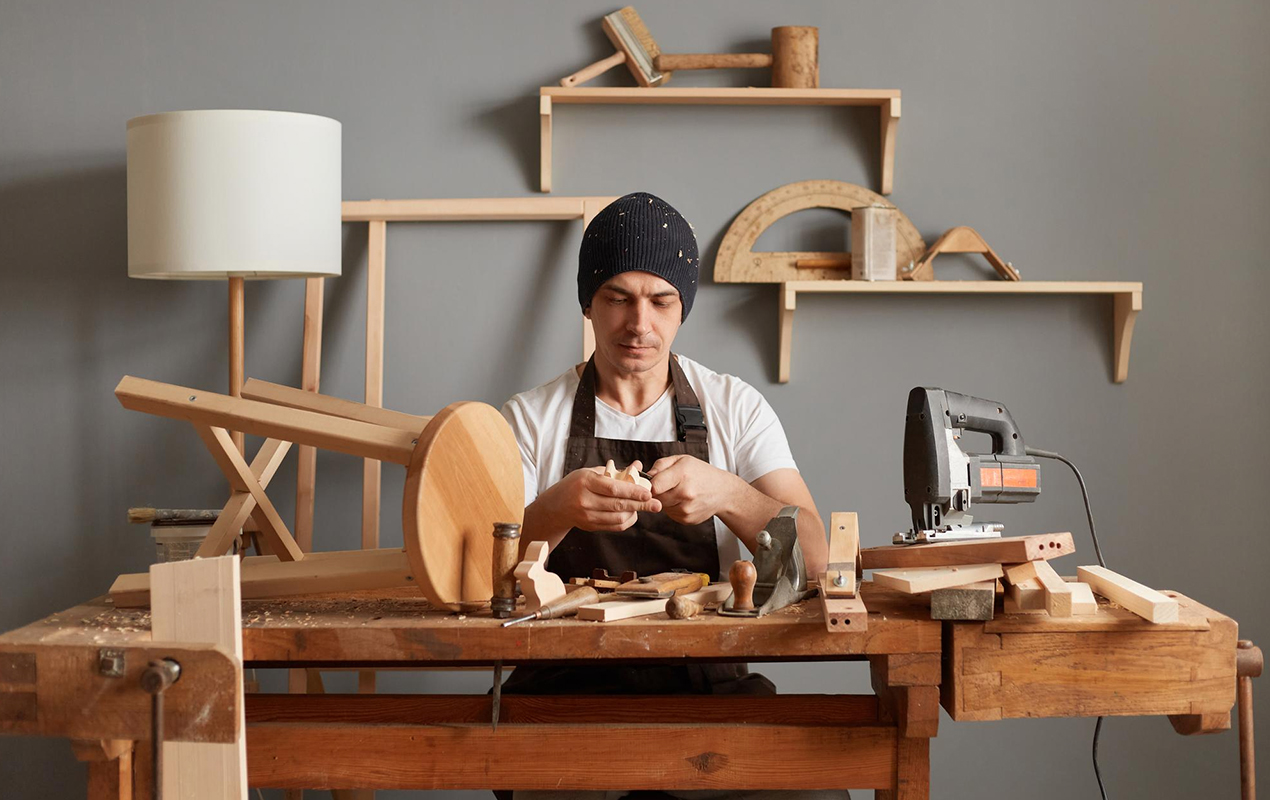The photograph captures a man working intently at a woodworker's table in what appears to be a decorative or mock-up studio setup. The setting features hues of gray and brown, giving a somewhat staged rather than practical appearance. The man, seated and facing the camera, is dressed in a white t-shirt, a brown apron, and a black beanie speckled with wood shavings. He is deeply focused on a piece of wood held in his hand, appearing to either study or carve it with a small tool. The table in front of him is cluttered with various wood pieces, including a stool turned on its side, chisels, planes, and a small wooden figure resembling a rabbit. To the right of the table is an electric saw, while a sander is positioned to his left. In the background, wooden shelves that seem too flimsy for a real workshop hold mallets, measuring tools, and other wooden items. A wooden lamp with a white cylindrical shade adds to the decor on the left side of the scene.